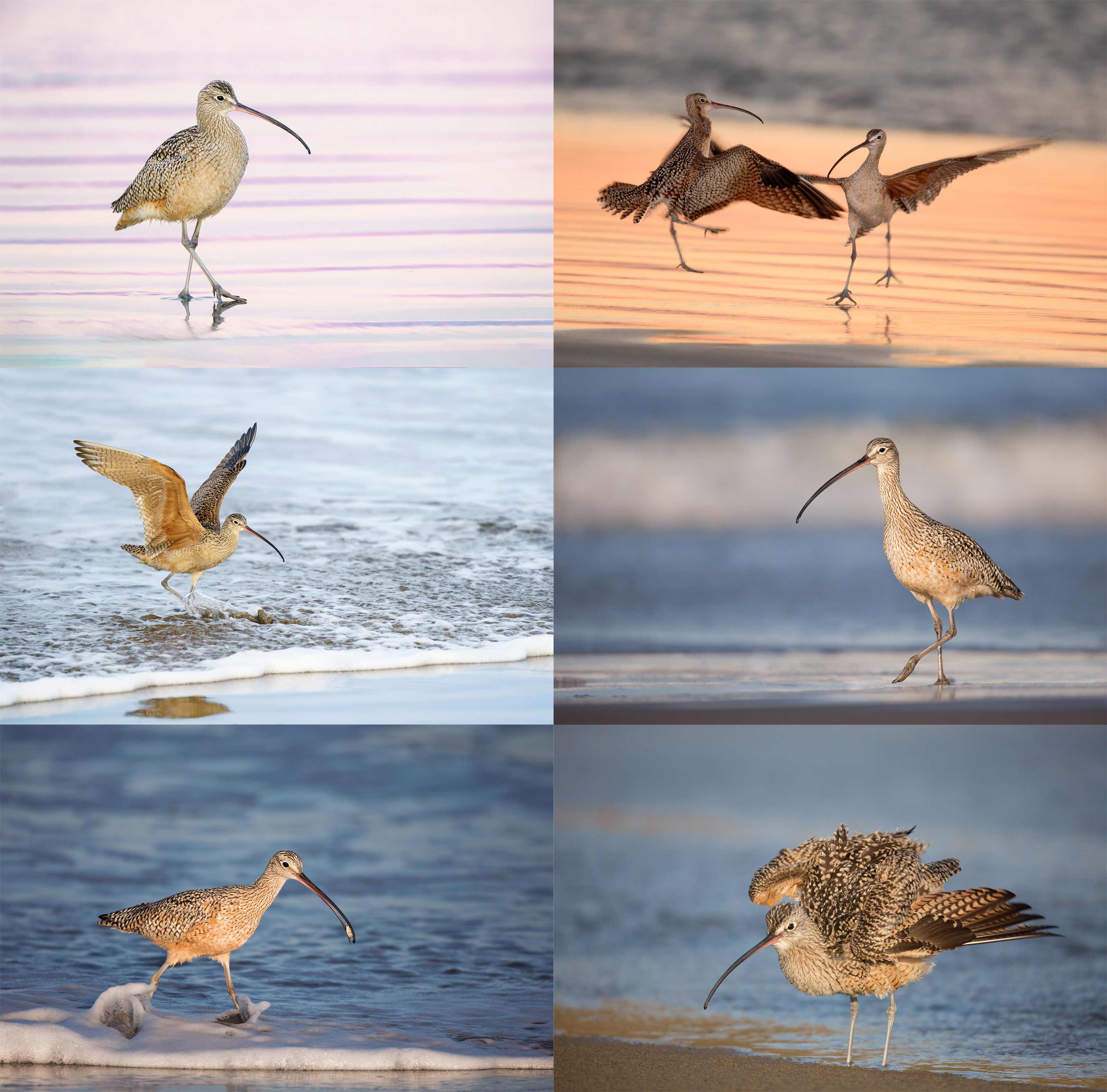The image is a collage of six photographs, all featuring a tan-colored seabird with brown speckles and a prominent, long, thin beak. The bird has long legs and is depicted in various activities along the seashore, with subtle differences in background coloration – pink in the top left and orange in the top right.

1. Top Left: The bird is seen walking along the shore with a pink background.
2. Top Right: Two seabirds are dancing around each other, set against an orange background.
3. Middle Left: The bird is attempting to pull a fish from the water, its wings raised as it stands in the waves.
4. Middle Right: The bird is walking on sand with a blurred background.
5. Bottom Left: The bird is wading through slightly deeper water, running with the ocean in the background.
6. Bottom Right: The bird, perched on the sand, has its wings extended.

Despite the variety of poses and activities, the bird's defining characteristics—its long beak and legs—are consistent across all images.